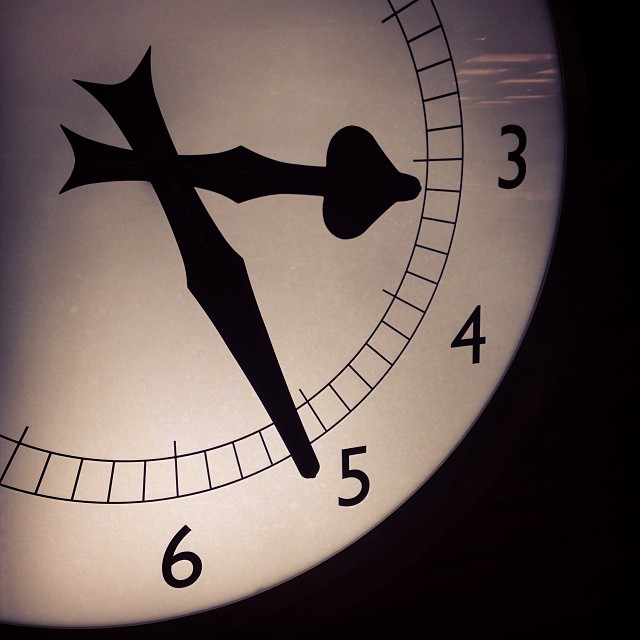This close-up photograph captures a partial view of a round clock set against a stark black background. The sleek, black frame of the clock blends seamlessly with the dark backdrop, giving it an almost floating appearance. The image focuses on a segment of the clock face, specifically from just above the three o'clock mark to just left of the six o'clock mark, showing the numerals three, four, five, and six clearly. The reflective surface of the clock reveals faint reflections of rectangular fluorescent ceiling lights, adding a subtle texture to the otherwise minimalistic composition. The clock's hour and minute hands, also black, are positioned within this visible portion, contributing to the overall monochromatic aesthetic.